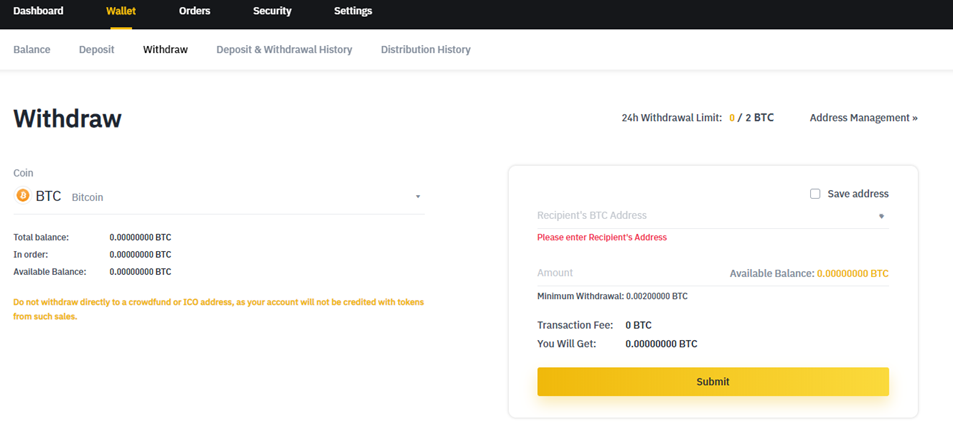### Detailed Caption for a Bitcoin Wallet Web Page:

This web page is an interface for a Bitcoin wallet. The top section features a black navigation bar with horizontally aligned options on the left: "Dashboard," "Wallet," "Order," "Security," and "Settings," all in bold white text. The "Wallet" option stands out in yellowish-gold, indicating it is the current selection.

Directly beneath this navigation bar is a submenu set against a white background, separated from the rest of the page by a gray horizontal line. The submenu includes the following options in bold gray text, from left to right: "Balance," "Deposit," "Withdrawal," "Deposit and Withdrawal History," and "Distribution History." The "Withdraw" option is highlighted in black, denoting the active section.

Below this submenu, the main body of the page displays the title "Withdraw." Following this, relevant details about the Bitcoin wallet are provided:
- **Coin:** Bitcoin
- **Total Balance:** 0.00 BTC
- **In Order:** 0 BTC
- **Available:** 0 BTC

At the bottom of this section, a cautionary note in gold text advises users: "Do not withdraw directly to a crowdfund or ICO address as your account will not be credited with tokens from such sales."

On the right side of the page, there is a panel displaying:
- **24-hour Withdrawal Limit:** 0 out of 2 Bitcoin
- **Address Management:** (Presumably, options for managing withdrawal addresses)

Beneath these details, there are input fields for the user to complete a Bitcoin withdrawal:
- A box to enter the Bitcoin address for the transfer.
- A field for the transfer amount, flanked by the available balance.
- Information on the maximum withdrawal limit.
- The applicable transaction fee and the net amount of Bitcoin to be received after the fee deduction.

This section concludes with a "Submit" button to finalize the withdrawal request.

Overall, the page is structured to provide a clear, step-by-step process for withdrawing Bitcoin, complete with important warnings and relevant financial limits to ensure secure transactions.